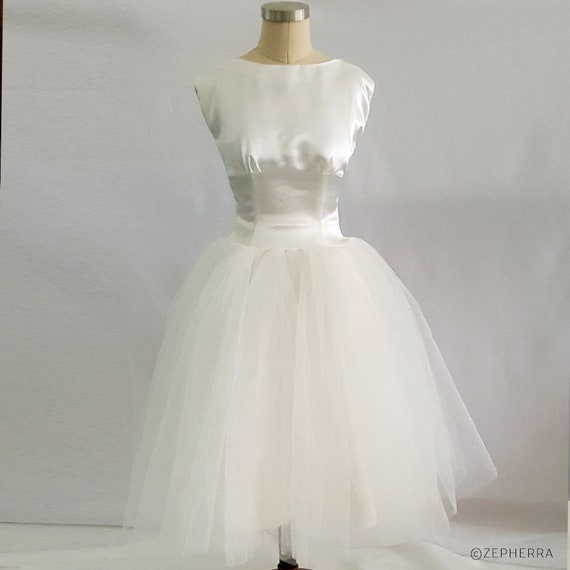This vertical rectangular photograph features a stunning, sleeveless white wedding dress displayed on a mannequin. The dress, crafted with layers of delicate mesh fabric that create a voluminous, tutu-like effect near the skirt, elegantly flares out from a cinched waistline adorned with a band. The bodice, made of a shimmering satin-like material, covers the shoulders and chest while showcasing an intricate mesh middle section. The mannequin, which has no arms, displays the dress from the neck down to the floor, touching the ground with its flowing layers. The background is a soft gray, giving a monochromatic atmosphere to the entire composition. Notably, the bottom right corner of the image bears gray lettering stating "Zephyra," attributing the design to this label. This wedding outfit exudes an ethereal charm, beautifully captured in a simple yet evocative setting.